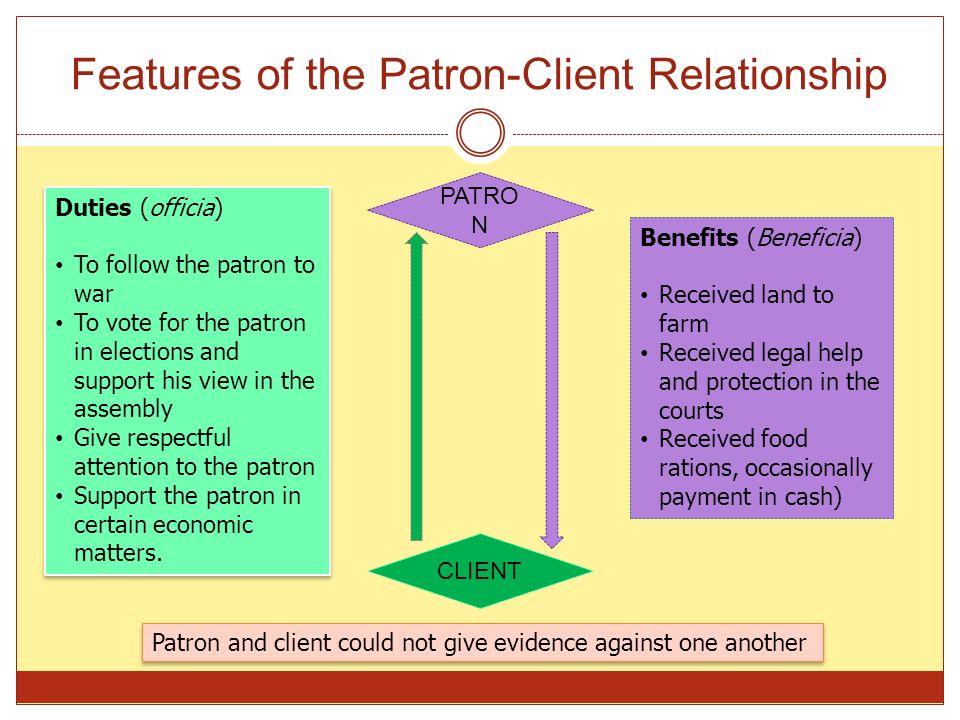The image is a detailed infographic titled "Features of the Patron-Client Relationship" in dark red at the top on a white background. The infographic is divided into three main sections: duties, benefits, and a mutual legal note at the bottom, all connected by a central diagram. 

On the left side, within a bright green box labeled "Duties (Officia)" with a drop shadow and a white border, are bullet points outlining the client's obligations:
1. Follow the patron to war.
2. Vote for the patron in elections and support his views in the assembly.
3. Give respectful attention to the patron.
4. Support the patron in certain economic matters.

In the middle of the infographic, a horizontal purple diamond labeled "Patron" is connected by arrows to a green horizontal diamond labeled "Client," symbolizing the reciprocal relationship. The purple arrow points from Patron to Client and the green arrow points from Client to Patron, denoting the mutual exchange of services and benefits.

On the right side, a purple box labeled "Benefits (Beneficia)" lists the patron's provisions to the client:
1. Receive land to farm.
2. Receive legal help and protection in the courts.
3. Receive food rations.
4. Occasionally receive payments in cash.

At the bottom, a pink box highlights a mutual agreement: "Patron and client could not give evidence against one another." This section is underscored by a horizontal red line on a yellow background, emphasizing the binding nature of this stipulation.